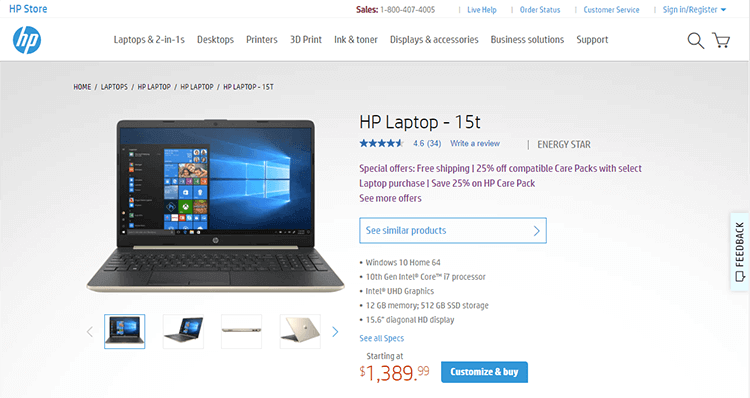This is a detailed screenshot of the Hewlett Packard (HP) website, captured from a desktop or laptop view. In the upper left corner, the iconic HP logo is prominently displayed—a blue circle with the letters "HP" in white. Just above the logo, "HP Store" is written in blue letters. 

Across the top of the webpage, a series of header titles provide navigation options: "Laptops and 2-in-1s," "Desktops," "Printers," "3D Print," "Ink and Toner," "Displays and Accessories," "Business Solutions," and "Support." On the far right side of the header, a magnifying glass icon indicates a search function, and next to it is a shopping cart icon.

At the very top of the webpage, there is a contact number for sales, prominently displayed with the word "Sales" in dark red font, and the phone number in black. To the right of the contact information, four sections are listed in blue ink: "Live Help," "Order Status," "Customer Service," and "Sign-In/Register."